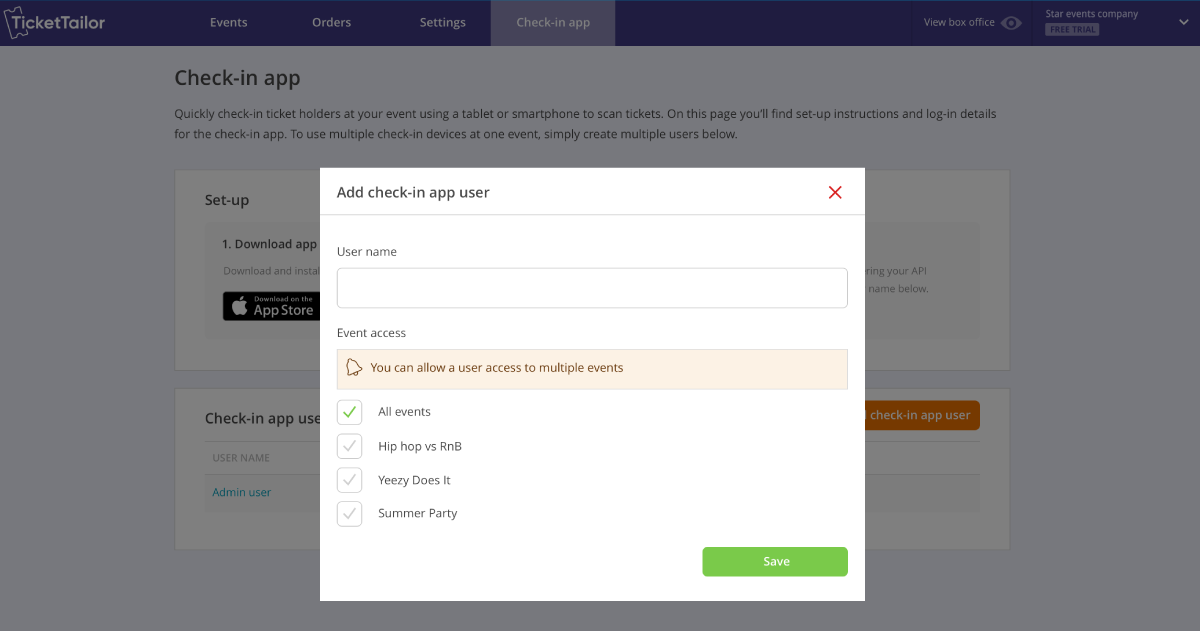The image features a user interface from the Ticket Tailor platform. The background is a dark blue, and at the top left is the heading "Ticket Tailor," accompanied by navigational tabs labeled "Event," "Orders," "Settings," and "Check In App." At the top right, there are options for "VIEW BOX OFFICE," "STAR EVENT COMPANY," and "FREE TRIAL." The "Check In App" tab is selected and highlighted in white.

Below the selected tab, there is a section with the title "CHECK IN APP" and a description that reads, "Quickly check in ticket holders at your event using a tablet or a smartphone to scan tickets. On this page, you will find setup instructions and login details for the Check In App. To use multiple Check In Devices at one event, simply create multiple users below."

Further down, there are buttons labeled "SETUP," "DOWNLOAD AN APP," and "CHECK IN APP USERS."

In the foreground, a white pop-up window with black text is displayed. The text on the pop-up reads "ADD CHECK IN APP USER," followed by fields for "USERNAME" and "EVENT ACCESS." Under "EVENT ACCESS," in brown text, it states, "YOU CAN ALLOW A USER ACCESS TO MULTIPLE EVENTS," and it includes checkboxes for "ALL EVENTS," "HIP HOP VS R&B," "EASY DOES IT," and "SUMMER PADS." The checkbox for "ALL EVENTS" is selected, which automatically ticks all other event checkboxes. At the bottom right of the pop-up, there is a green button labeled "SAVE."